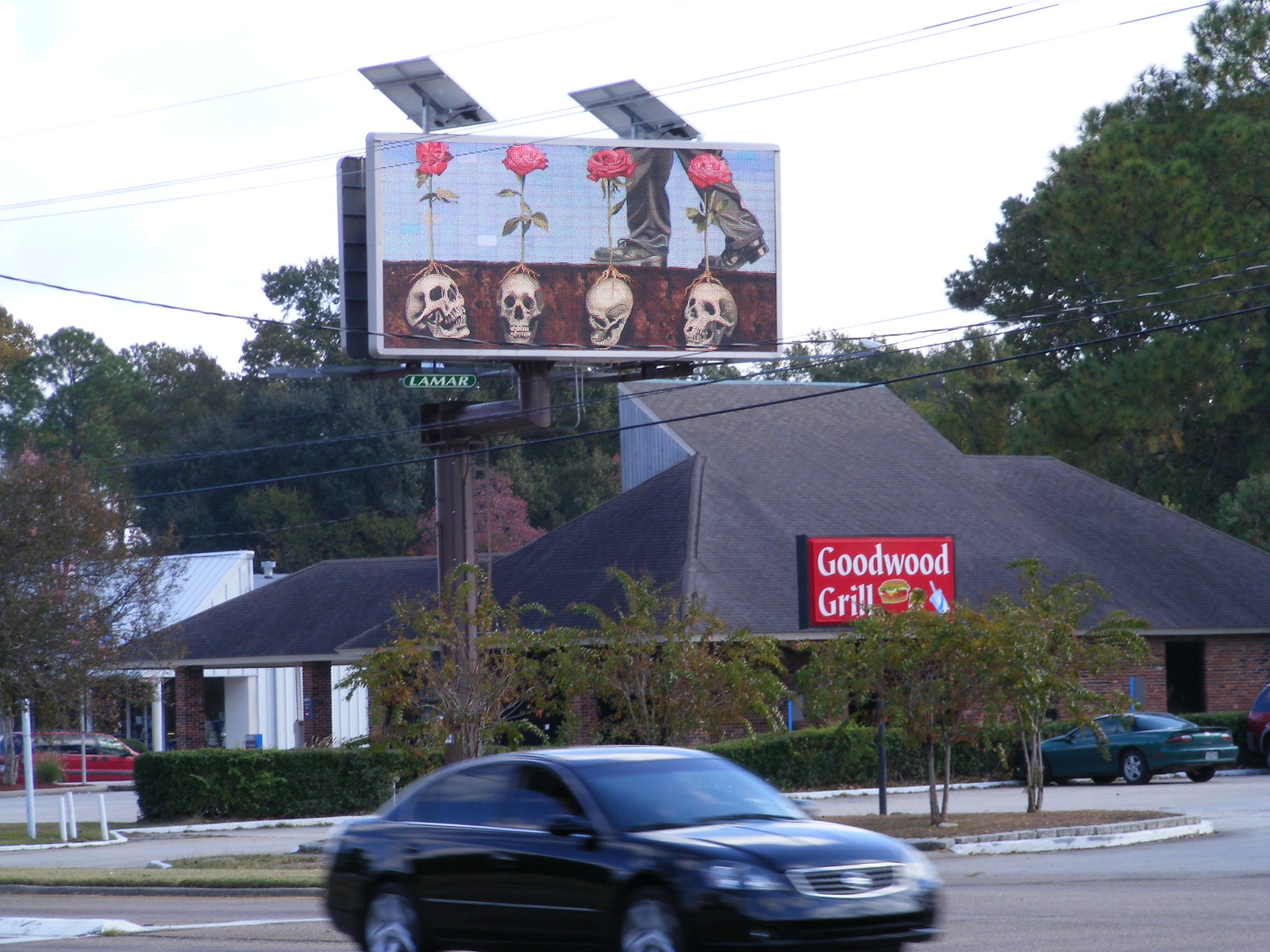This vibrant outdoor photograph captures a dynamic street scene. Central to the image is a sleek black Nissan driving past a similarly black four-door vehicle. In the lower right corner, a green late-90s model Camaro is parked, adding a nostalgic touch. The background features a prominent red sign with white letters that reads "Goodwood Grill," accompanied by an enticing image of a burger and soft drinks. Above this sign is an eye-catching billboard displaying a surreal artwork: blooming roses intertwined with human skulls at their base, each skull distinctively positioned—with one looking up, another looking ahead, a third gazing down and to the right, and the fourth staring to the left. The scene is framed by lush green trees and intersected by power lines, giving it a quintessentially urban feel.